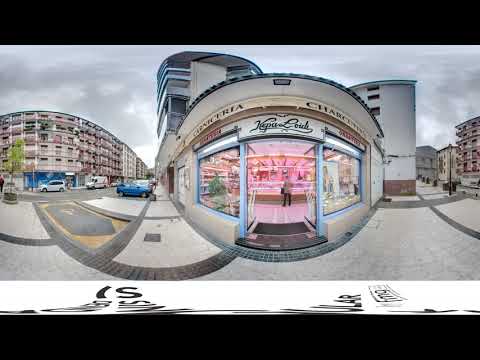The image appears to be a panoramic, possibly distorted through a fisheye or some filtering lens, depicting an outdoor urban setting with a distinct confectionery shop at the center. The shop interior is visibly pink, with pink lighting or displays, and shows a person standing at a counter with their back to the viewer. The shop is part of a building complex featuring an oval-shaped structure to the left, identified as an apartment building, surrounded by multiple cars. To the right, the street is devoid of cars and is flanked by additional multi-story buildings, including one pinkish in color and another beige. The scene includes a tree in front of the pink building and a pathway running alongside. Distorted text can be seen at the bottom of the frame, with letters resembling "A", "R", and "S". The photograph, taken during an overcast day, presents vivid colors including bright pink, light blue, black, gray, silver, maroon, dark blue, brick red, and brown, adding to its vibrant depiction of downtown life.